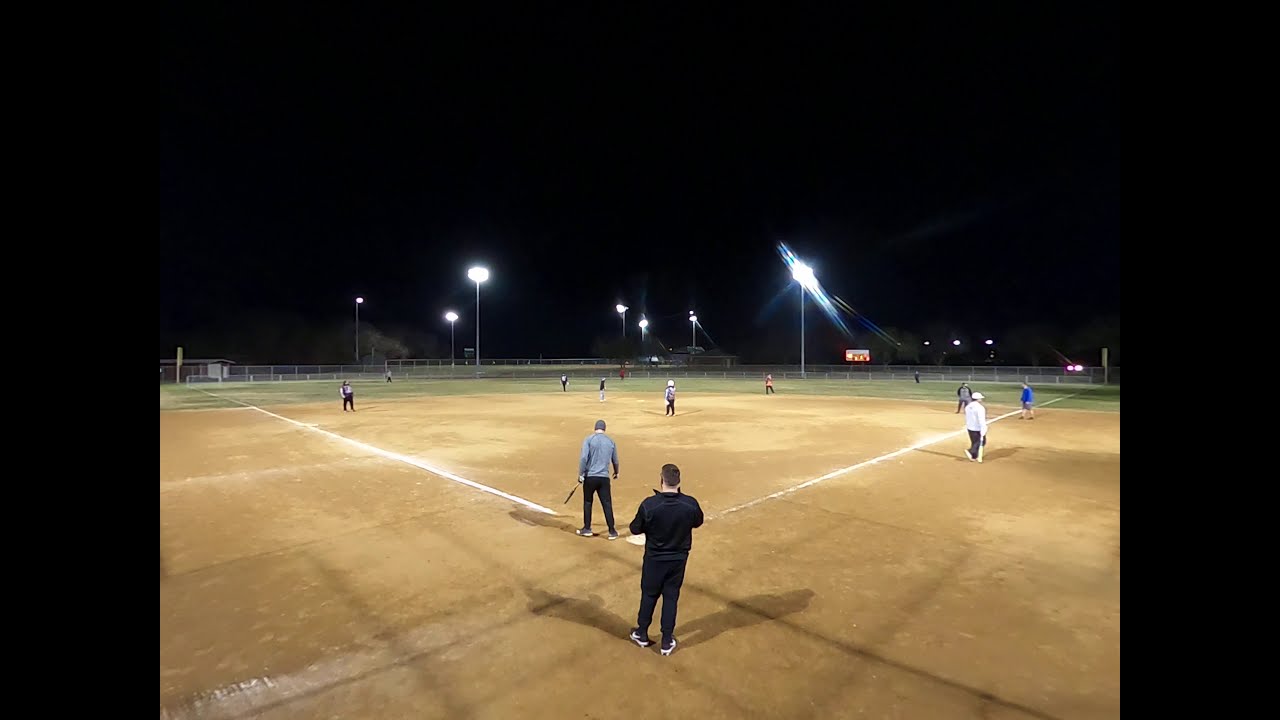The nighttime scene captures a lively co-ed softball game on a well-lit sports field. The image has a large black border on both the left and right sides, focusing the viewer's attention on the action. The central focus is on a man in black attire, standing ready to catch the incoming ball, while a batter in gray top and black pants adjusts his stance at the plate. Other players are scattered across the expansive field, including a woman pitcher preparing to throw. The well-maintained field is characterized by dusty dirt and clearly marked white chalk lines. The distant background features faint outlines of a scoreboard and surrounding fencing illuminated by strategically placed light poles, contrasted against the dark night sky.